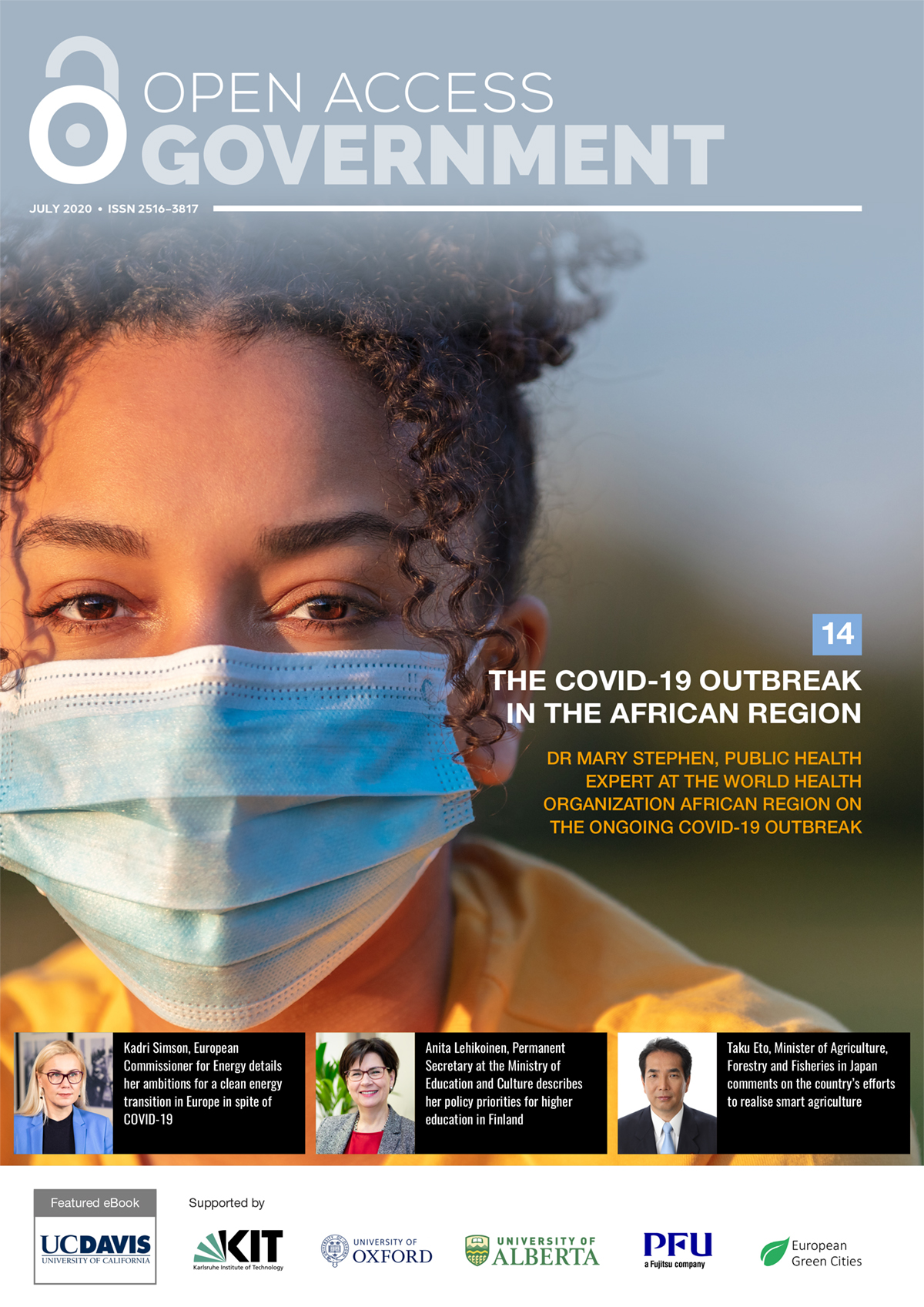**Open Access Government - July 2020 (ISSN 2516-3817)**

The cover features a striking photograph of a Black woman with very curly hair styled up, with tendrils framing her face. She is wearing a blue paper face mask that covers her mouth and nose, and her expressive brown eyes look directly at the viewer. She is dressed in an orange shirt or jacket, which adds a vibrant contrast to the slightly out-of-focus background.

In the foreground, a prominent unlocked lock symbol accompanies the text "Open Access Government." Below this, the title "July 2020 ISSN 2516-3817" is displayed.

To the right, a blue square with the number "14" introduces an article in orange text about the COVID-19 outbreak in the African region. The article is authored by Dr. Mary Stephan, a public health expert at the World Health Organization African Region, detailing the ongoing COVID-19 outbreak.

Below this feature are three profile images accompanied by their respective details:

1. A white woman with blonde hair, wearing a blue jacket and glasses, identified as Kandri Simmons, the European Commissioner for Energy, discussing the details and missions for a clean energy transition in Europe despite COVID-19.

2. Anita Lehikoinen, the Permanent Secretary at the Ministry of Education and Culture, who elaborates on her policy priorities for higher education in Finland.

This detailed cover sets the stage for an insightful edition focused on pivotal health, energy, and education issues amidst the pandemic.